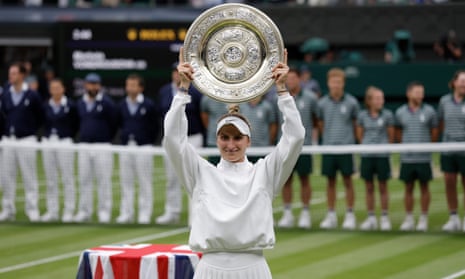The image captures a celebratory moment on a grass tennis court, where a professional female tennis player, dressed immaculately in white including a visor, stands prominently in the foreground. She proudly holds aloft the iconic Wimbledon trophy, a decorated circular silver platter with intricate engravings and golden accents. Beside her, a round table draped with a red, blue, and white tablecloth bearing the British flag adds a touch of ceremonial splendor. The meticulously mowed grass surface, with its alternating light and dark stripes, enhances the scene's visual appeal. In the background, a tennis net separates the player from two groups of onlookers, presumably officials and ball boys. On the right, older individuals dressed in white pants and dark blue shirts stand neatly in a row. To the left, a younger group, likely the ball catchers, are attired in dark shorts and blue and white striped shirts with white shoes. Further behind, a scoreboard with gold lighting and a crowd of spectators, some shielding themselves with green umbrellas from a light drizzle, complete the backdrop of this triumphant awards ceremony.